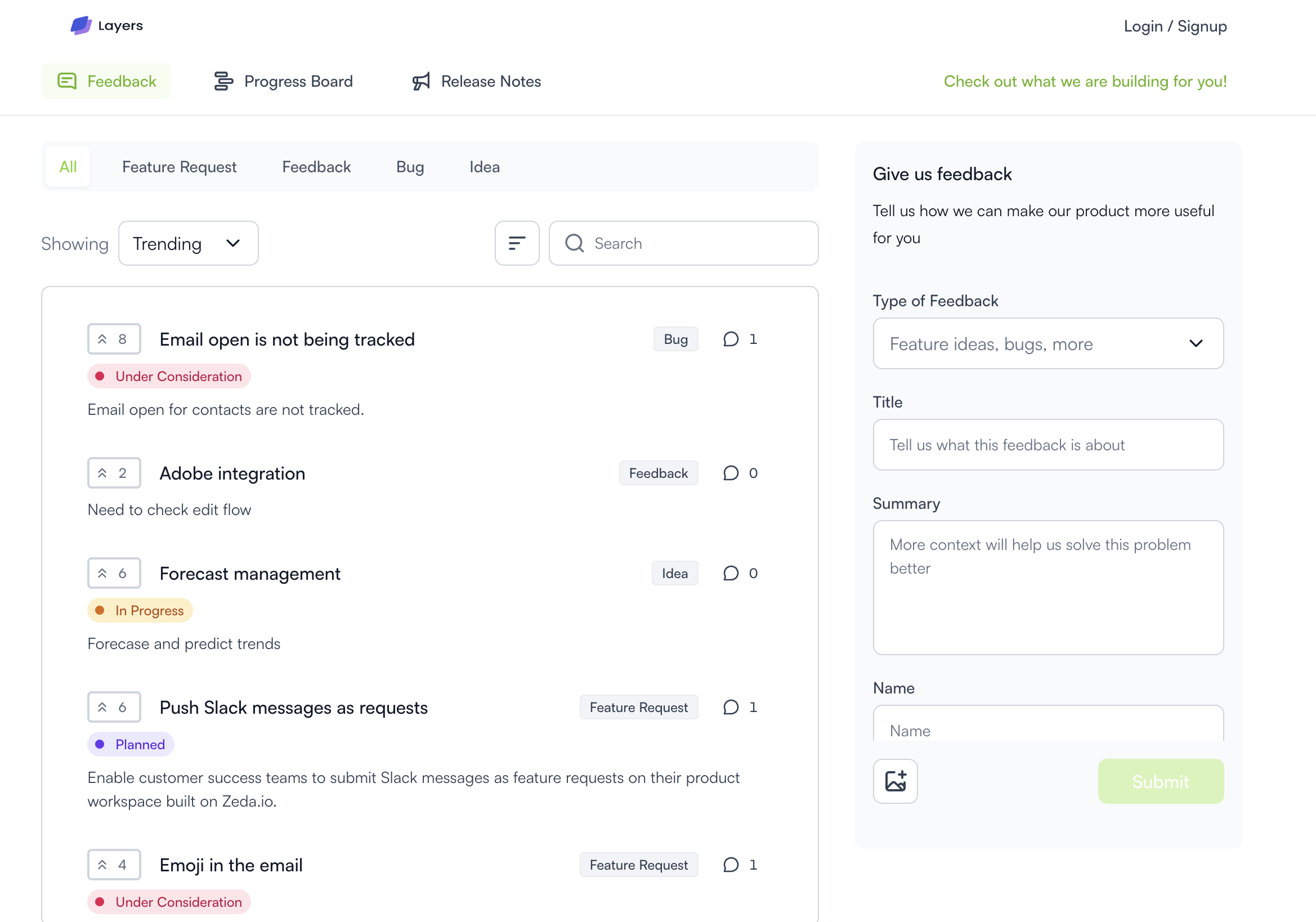Here is a detailed and cleaned-up caption for the image described:

---

In this image, we see a webpage or application interface named "Layers." The logo, featuring the word "Layers" in black text, is positioned in the top-left corner. There are two overlapping squares—one blue and one purple—hovering beneath and over each other beside the logo. 

In the upper-right corner of the page, there are "Login" and "Sign Up" buttons. Below the logo on the left side, there is a menu with options including "Feedback," "Progress Board," and "Release Notes." 

On the right side, prominently displayed in green text, is a message saying, "Check out what we are building for you." 

Near the top-left area, there are several tabs labeled "All," "Feature Request," "Feedback," "Bug," and "Idea." Beneath these tabs, there is a drop-down menu, followed by a search box and a search icon.

Further down, there is a section titled "Give Us Feedback" on the right side. At the top of this section, it reads, "Tell us how we can make our product more useful for you." There is also a drop-down box for selecting the type of feedback, along with fields for a title and a summary to enter detailed feedback.

Between these sections is a box-like outlined window listing various features and integrations such as "Email Open is Not Tracked," "Adobe Integration," "Forecast Management," "Push Slack Messages as Request," and "Emoji in the Email."

---

This caption provides a clear, structured, and comprehensive description of the image, incorporating all the mentioned elements in an organized manner.